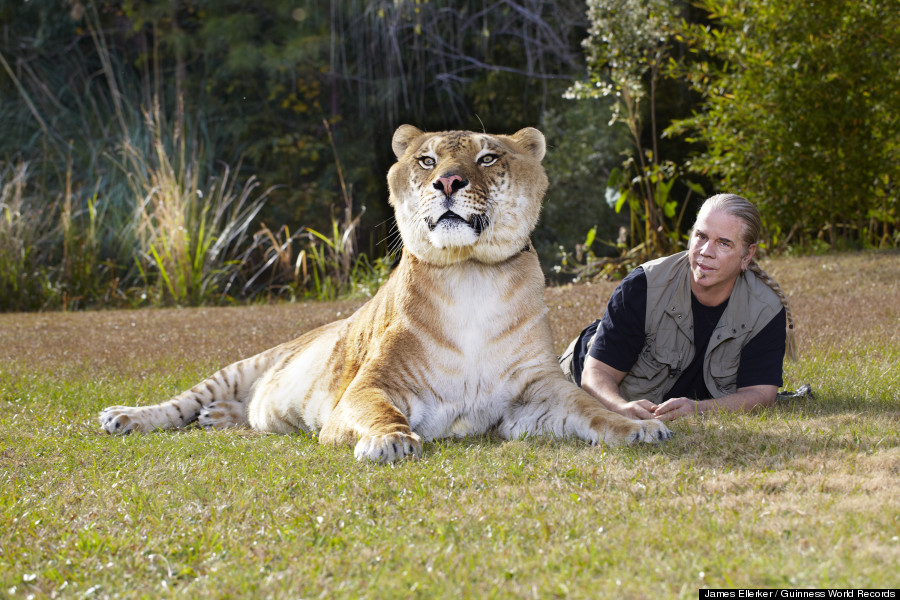In a sunlit jungle-like area, a man with a ponytail braid and tan skin lies relaxed on short green grass, wearing a black shirt and a khaki-gray vest. Beside him lies an exceptionally large lion with an unusual coloration of white, yellow, and brown fur, a prominent pink nose, and greenish eyes. The lion, which has a notably large head and chest, appears calm and is looking distantly alongside the man. Both are surrounded by abundant greenery, including shrubbery, yellow hues, and patches of brown from the terrain and plant life. The backdrop features a combination of tall grasses, possibly bamboo, and leafless deciduous trees, giving the scene a wooded, secluded feel. In the bottom right-hand corner of the image, text in white on a black background reads, "James Ecker, Guinness World Records," underscoring the extraordinary nature of this serene encounter.